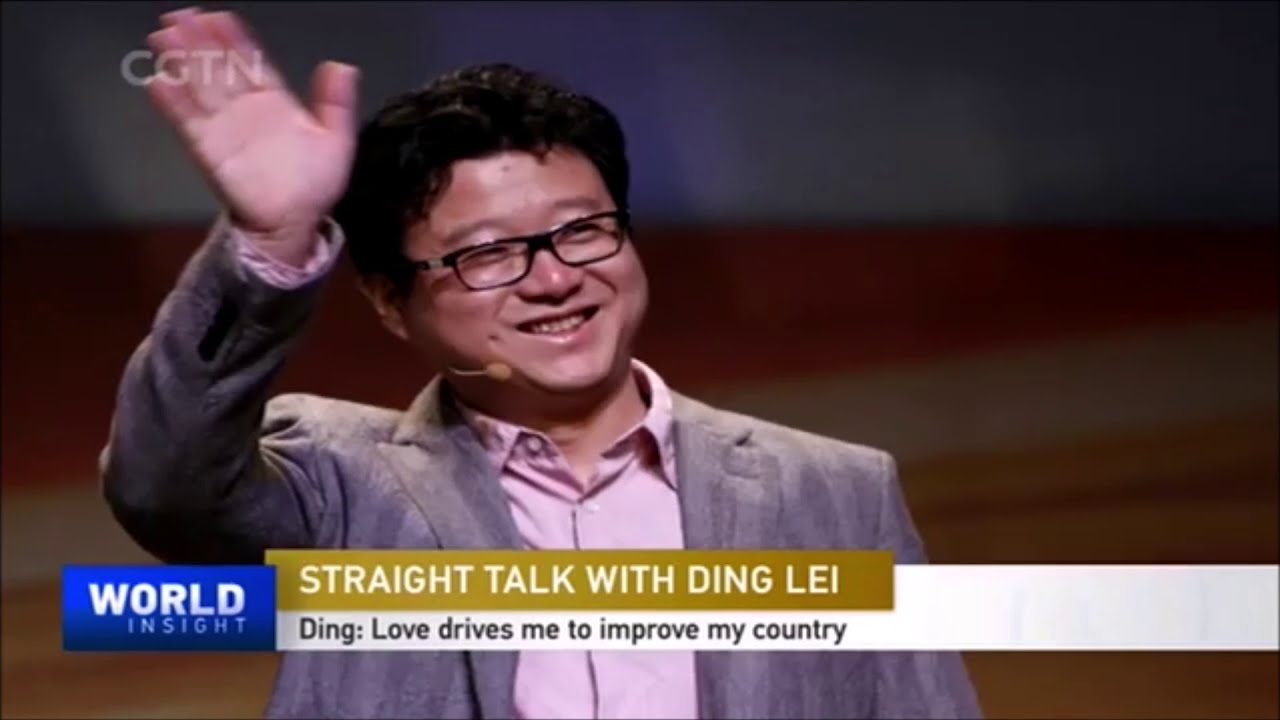The image depicts a television screenshot featuring an Asian man positioned at the center-left, cropped at the waist. He is wearing a gray blazer over a light pink button-down shirt and black-framed glasses. His hair is short, dark black, slicked back with volume, and he has a small, light gray to yellow microphone attached to his left ear. The man, identified as Ding, appears to be in mid-wave with his right arm raised, smiling and looking slightly to his right. 

In the top-left corner, the watermark "CGTN" is visible in light gray text. A blue banner at the bottom-left displays the white text "World Insight," with "World" in a larger font than "Insight." Adjacent to this banner is a gold rectangle containing the white text "Straight Talk with Ding Li," followed by a black text caption below that reads, "Ding: Love Drives Me to Improve My Country." The background appears dark, emphasizing the central figure and the on-screen text.